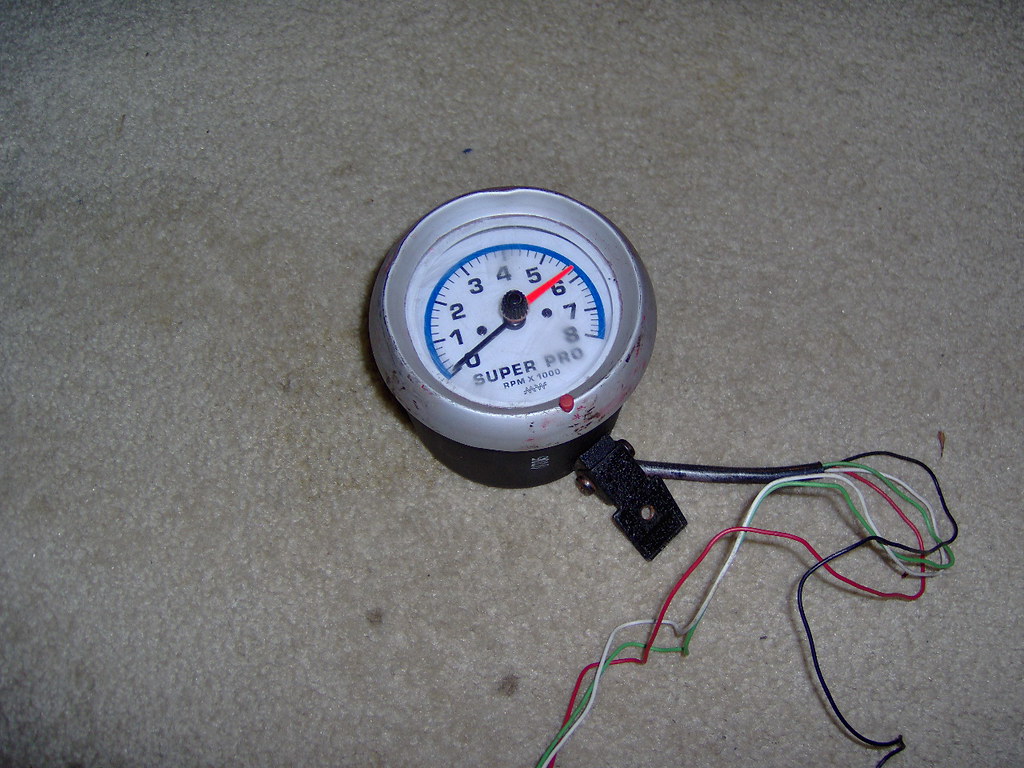The image depicts a metallic grey gauge, likely a tachometer, resting on a surface that could either be the floor, possibly tile, or a table. The device features a black backing and a front display with a blue line marking the tachometer scale, which ranges from 0 to 7 (0, 1, 2, 3, 4, 5, 6, 7). The display includes the text "SUPER PRO RPM x1000" written in black ink. The gauge has two indicator hands: one black and one red, pointing in opposite directions. Visible at the back of the gauge are several colored wires: black, red, white, and green.